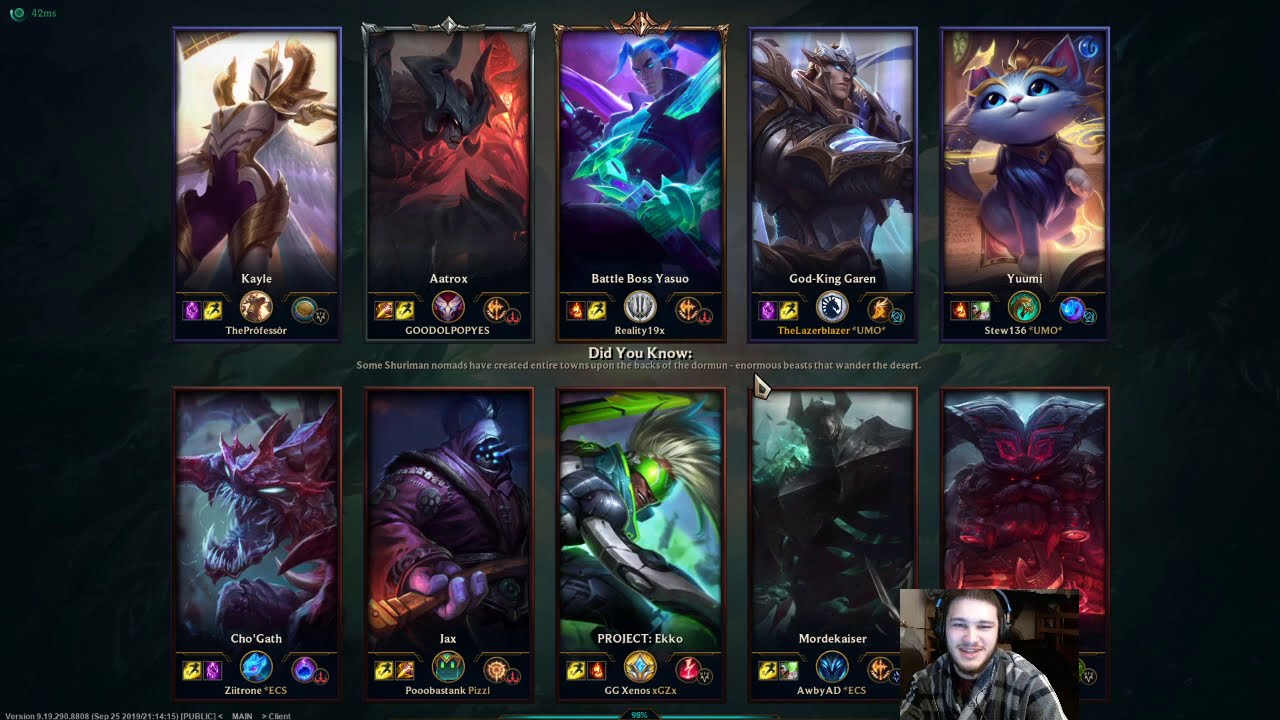In this detailed screenshot from a video game interface, the backdrop is predominantly black, highlighting a small emblem in the upper left-hand corner with the number "42" in green, followed by "MS". The bottom of the screen features tiny, hard-to-read white text. In the bottom right corner, there is a video capture of a young white male with a mustache and a slight beard, wearing headphones and a plaid shirt. He is showcasing his screen to viewers, where a grid of ten intricate and colorful cartoon-esque video game characters is displayed, arranged in two rows of five. 

The first character in the top left is a female warrior clad in full armor. Next to her is a balrog-like figure with a menacing appearance. The third character is a cartoon male with blue hair, wielding a sword. Adjacent to him is another male character, donned in gray and gold armor with a helmet featuring wing-like designs. The fifth character on the top row is a fantasy cat dressed in clothes.

On the bottom row, the first image depicts a dragon-like creature. Next to it is a heavily armored warrior, while the third character is a man with a tall mohawk. The fourth character appears part-man, part-creature, contributing a blend of horror and fantasy to the lineup. The final character on the lower right looks like a monstrous entity with a lava-like body and prominent horns. This detailed assembly of fantasy and science fiction characters adds a layer of immersive depth to the gaming experience being shared by the player.